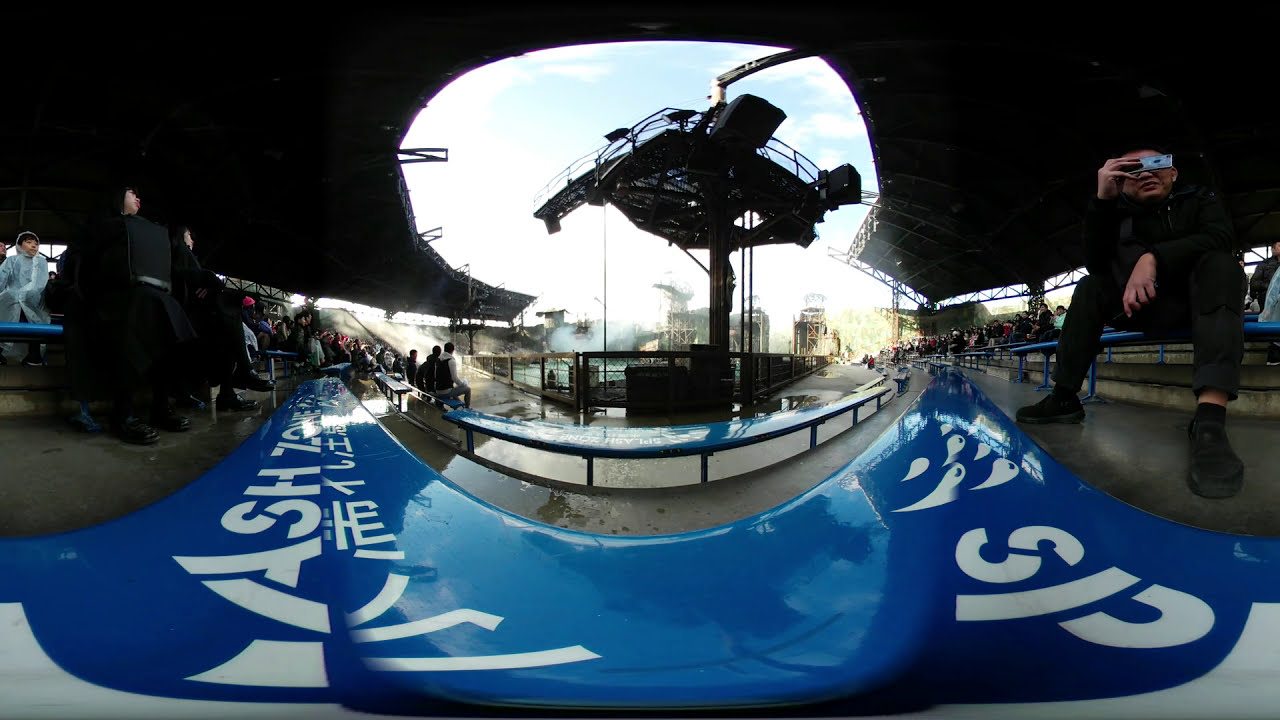This detailed panoramic, fisheye-lens shot captures a futuristic scene in a covered stadium arena with open skies and clouds in the backdrop. In the center, there’s an unidentifiable structure resembling a football field, potentially serving as a stage or some form of a sci-fi object anchored into the ground. On the right, a man dressed entirely in black, possibly an older white man, sits on a blue bench and is focused on taking a picture, holding a camera or phone to his face, obscuring his features. You can see his black shoes and slacks, and his outfit contrasts with the white text "SP" and "ASH" visible on a large, possibly metallic object in the foreground, which could be a vehicle hood or a jump ramp. People, seated and standing, clothed predominantly in dark attire, populate the background, all intently overlooking the primary area. The panoramic curvature of the image emphasizes the extensive seating area resembling bleachers, and the fisheye effect gives the scene an enveloping, immersive feel, as if taken with a 360-degree camera.